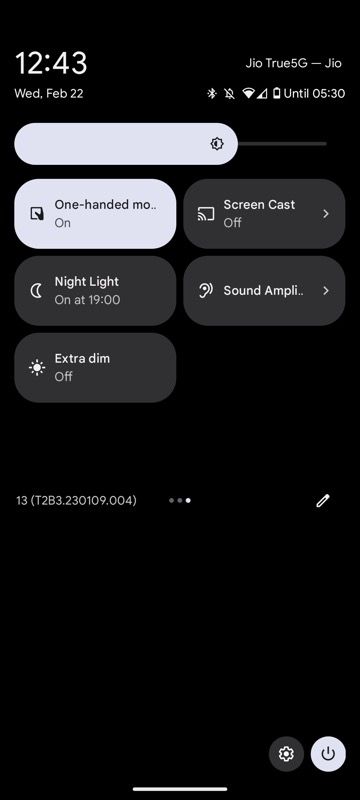An image of a mobile device settings screen set against a black background. In the top left corner, the time is displayed in white as "12:43." The date, "Wednesday, February 22nd," is shown below the time. In the top right corner, the status bar reads "Geo true 5G" beside several icons including Bluetooth, ringer (silenced), Wi-Fi, cell signal, and battery percentage, which indicates "until 5:30." The screen brightness slider shows brightness set at approximately two-thirds.

Below the status bar, various setting toggles are visible:
- "One hand mode" is on
- "Screencast" is off
- "Night light" is scheduled to turn on at 19:00
- "Sound amplifier" 
- "Extra dim" is off

Farther down, a line of text includes a code "13" with additional coding elements to the right, next to a pencil icon. At the bottom of the screen, there's a settings gear icon beside a white power button.